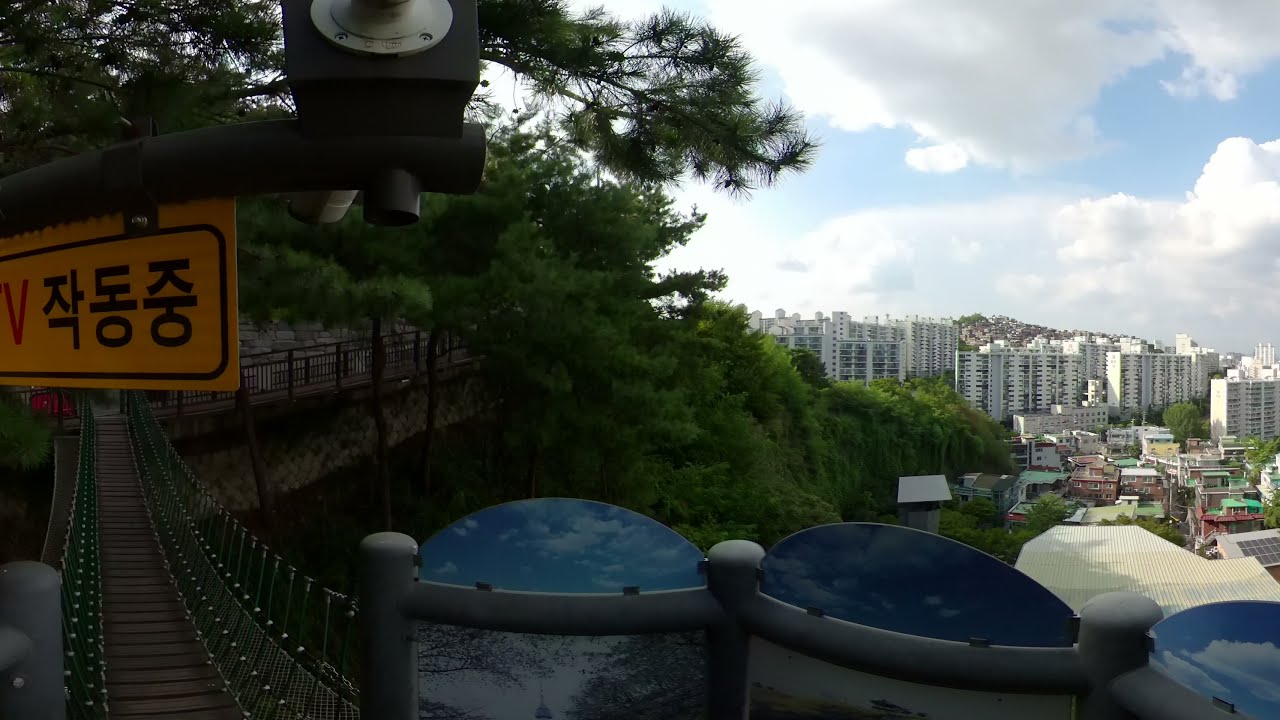This photograph captures a vibrant, multi-layered cityscape likely in Korea. The central focus is a picturesque suspension bridge on the left, made of brown wooden planks with green and brown railings and ropes, stretching over a ravine and flanked by lush green trees and shrubs. Above the bridge hangs a yellow sign with Korean characters, hinting at the location. The view from the higher vantage point reveals a blend of natural and urban elements. Towards the right, the cityscape unfolds with an assortment of white high-rise buildings, possibly hotels or apartments, adorned with numerous windows. Interspersed among these are smaller, colorful buildings—some brown, blue, green, and red—creating a dynamic visual palette. The backdrop features a mountainous area with additional houses dotting the slopes. An expansive, soft blue sky with fluffy white clouds enhances the overall serene yet bustling atmosphere of the city.